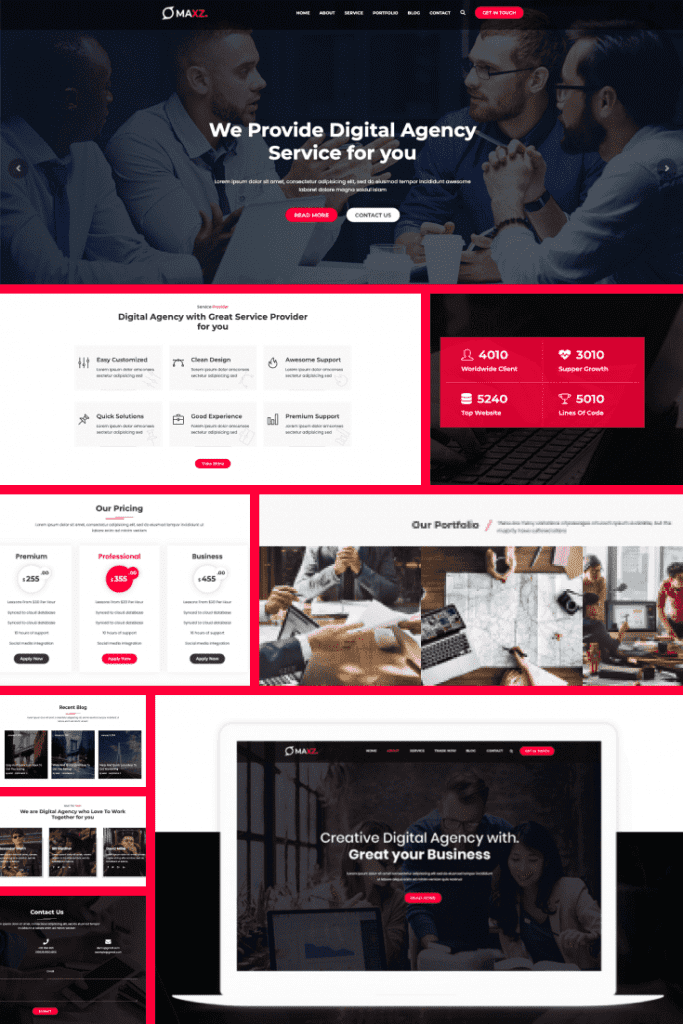The image is a screen capture of a website, which features a somewhat blurry top section with a partially legible red and white logo, a circular icon, and clickable white sub-menus, along with an apparent search box. Below this header, a red and white box is visible, followed by a prominent central image with the tagline "We provide digital agency service for you" in white text. Beneath the tagline, there's a brief description also in white text. 

The main image depicts a formal meeting setting with four men dressed in suits, two of whom are wearing glasses. They are seated at a table, engaged in a discussion, with an open laptop positioned in front of one of the men. 

Directly below this, two additional images can be seen. The first one, predominantly white with a black header, states "Digital agency with great service providers for you" followed by six smaller black blurbs, each accompanied by small icons. Adjacent to this is a red and white box containing statistics represented by icons, listing four different metrics.

Further down, there is another box, composed of red, black, and white sections, labeled "Our Pricing," though the exact text is too small to decipher. Adjacent to this are several photographs under the heading "Our Portfolio." These images include a man sitting at a desk, a person working on a laptop, a map spread out on a table, and a group of people gathered around a computer. 

Finally, at the bottom, there are about six smaller images featuring white text overlays. One black blurb with white text stands out, alongside an image of what seems to be a simulated laptop screen displaying the text "Creative Digital Agency with great your business." In the final scene, a man and a woman are seen collaborating on work around a table.